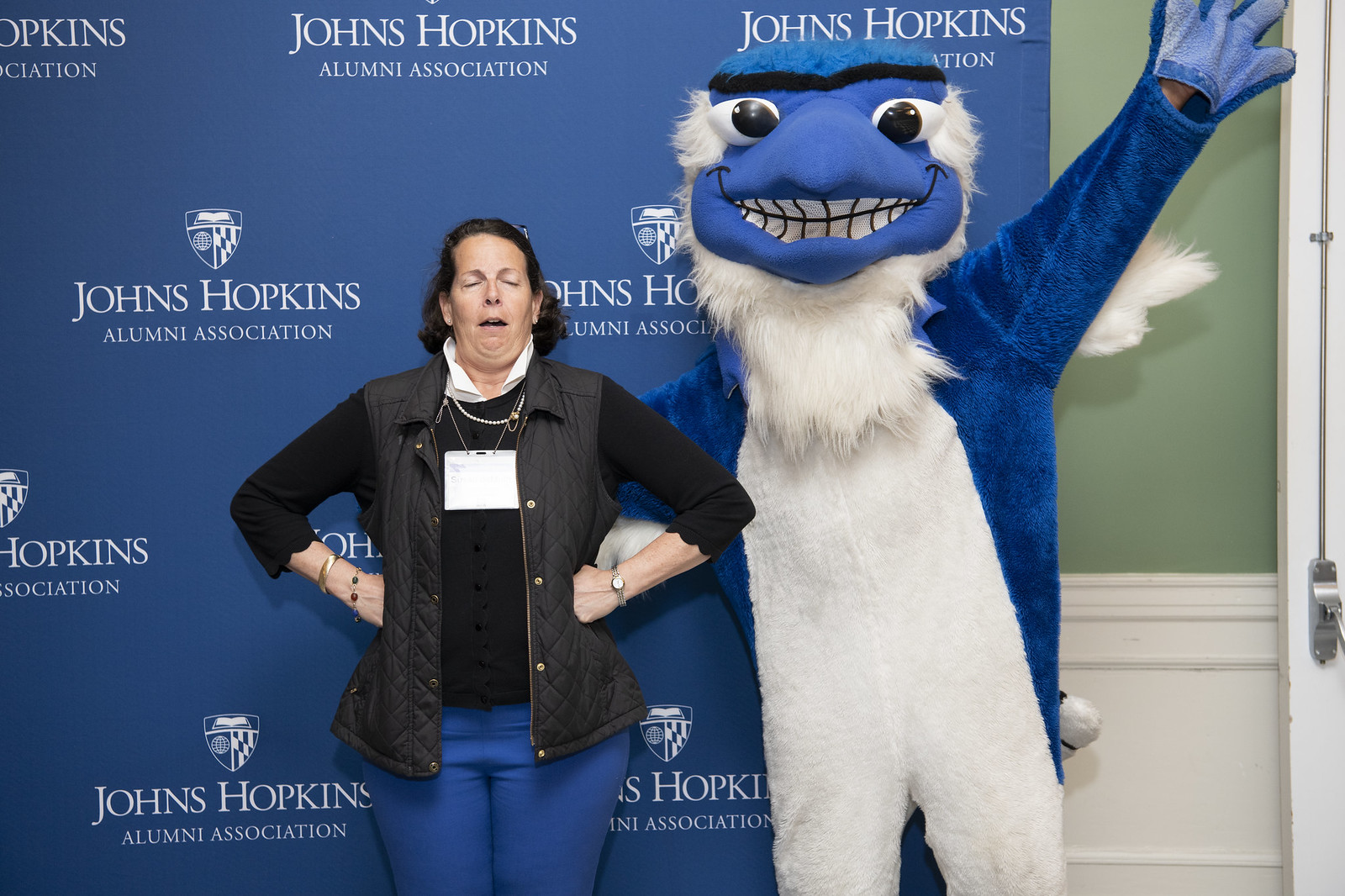In this image, a woman with short brown hair, dressed in a long-sleeved black shirt layered under a gray vest and paired with blue pants, stands with a humorous expression—eyes closed and mouth slightly open. She has both arms bent at the elbows, placing her hands on her hips, with a watch on her left wrist and bracelets on her right. Around her neck, she wears a necklace and a white name card that drapes down her chest. Next to her on the right is a mascot that resembles an eagle. The mascot is clad in a blue and white costume: a blue face with black eyebrows, beady black eyes, white fur around the face and neck, a white belly, and blue arms ending in blue gloves. The mascot’s left arm is extended outward, while the right arm wraps around the back of the woman. Behind them is a large blue banner with the words "Johns Hopkins Alumni Association" in white, alongside a shield logo, all set against a background wall that is green on top and white on the bottom.